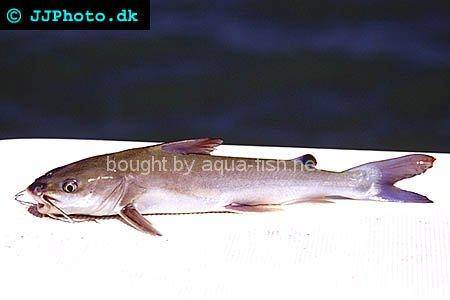This image depicts a fish, likely a catfish, characterized by its long whiskers, forked tail, and a mix of dark brown and grey hues atop its body, transitioning to a whitish underbelly. The fish appears to be approximately a foot long and is placed on a white surface, with its mouth open and one slimy eye visible. The background is murky and somewhat indiscernible, potentially featuring water or plants with elements of green and blue, as well as some purple lines. The top left corner of the image features a black rectangular strip with the text "jjphoto.dk" in a teal, four-year news style font, accompanied by a copyright symbol. The image background includes a blur that contains greenish elements, which adds to the overall muddy and undefined scene behind the well-focused fish.